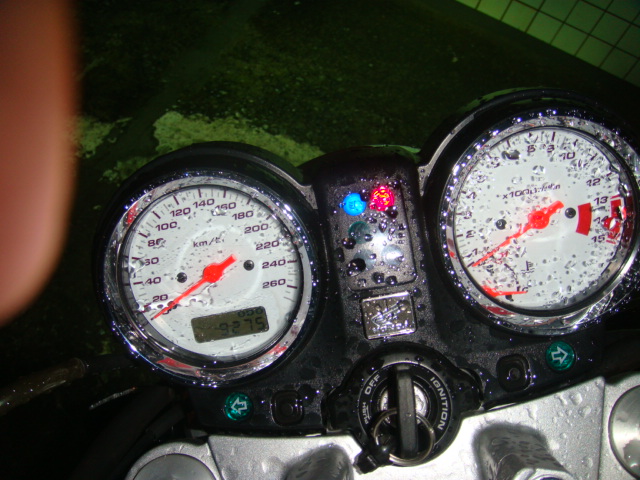This photograph features a close-up, overhead view of a pair of motorcycle handlebars, prominently displaying two dials adorned with raindrops. Below the handlebars, the background is ambiguous, showing either green grass or a dark-colored rug. In the top-right corner of the image, there are small tiles arranged at an angle.

The left dial is a large speedometer labeled "KM/H," featuring a red needle. Its scale ranges from 0 to 60, with numerical markings at increments of 20 (i.e., 0, 20, 40, 60), and smaller tick marks denoting individual units. There is also a rectangular LCD display at the bottom of this dial, showing the number "9275."

The right dial, possibly a tachometer, has a scale from 0 to approximately 15, marked with the term "times 100." Additional text is illegible. The intricate detailing of the dials, combined with the raindrops, creates a visually engaging and dynamic composition.